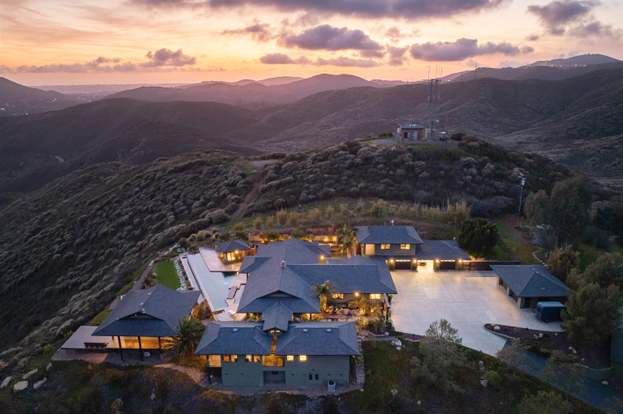The photograph captures a serene and somewhat secluded property set amidst rolling desert hills and surrounded by a distant backdrop of purplish mountains under a setting sun. The sky is painted in shades of gold, pink, and a light orange, accentuated by puffy clouds. Central to the scene is a large house with slate blue rooftops, flanked by several smaller buildings which share the same roof color. The property appears expansive, featuring a big driveway and significant open cement areas, possibly for parking or gatherings, and it exudes an air of wealth. A distinctive tower, perhaps for cellular connectivity, stands atop a hill behind the buildings. The landscape includes patches of green shrubbery, and a vast white area lies between some of the structures, further highlighting the sprawling nature of the estate. The overall ambiance is tranquil and picturesque, enhanced by the soft light of the setting sun, making it seem like an ideal spot for a vacation resort or an opulent retreat.